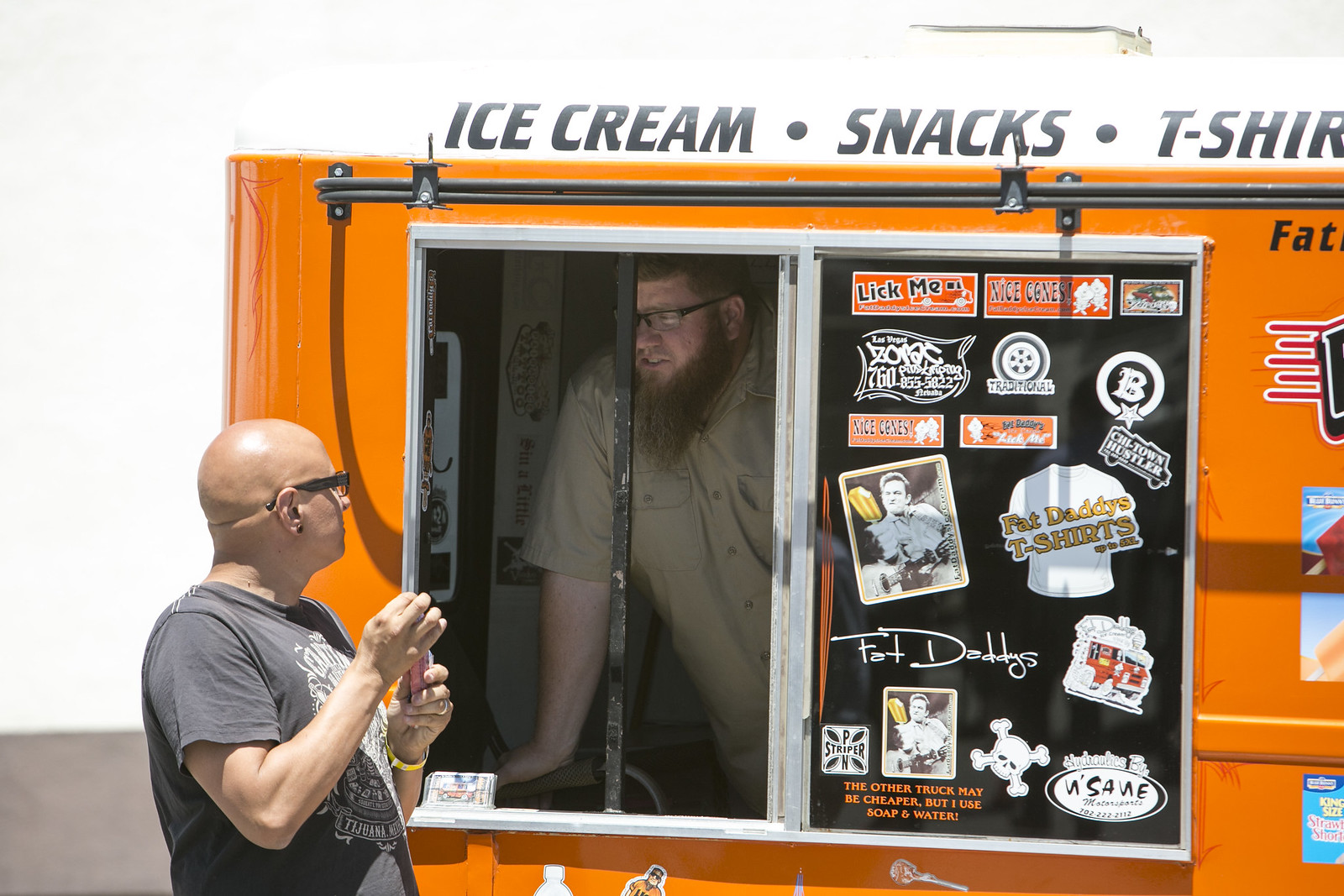This photograph depicts a vibrant scene of a man outside an eye-catching bright orange food truck, distinguished by its signage reading "Ice Cream, Snacks, T-Shirts" in black lettering on a white background. The man standing outside is bald, wearing black glasses and a black t-shirt with a white symbol on the center. He has his hands positioned in front of his chest as he engages in conversation with the truck operator. Inside the food truck, towards the right, stands a bearded man with short red hair, donning a beige short-sleeved button-down shirt and black glasses. He is leaning on the truck’s counter with his arms for support. The truck's window frame is silver metal with a central black metal bar. Surrounding the window are numerous colorful decals and product items, including stickers and a soccer jersey, adding to the lively and bustling atmosphere of this roadside exchange.